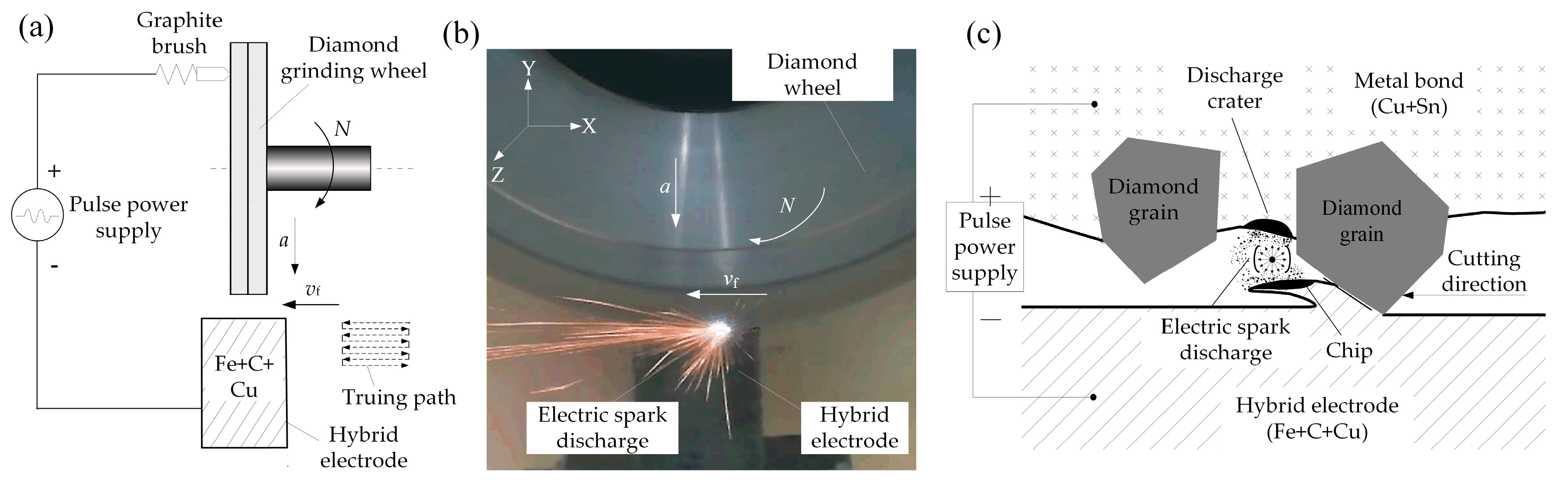The image is a comprehensive scientific diagram illustrating the process and specifications of a diamond grinding wheel mechanism, labeled A, B, and C. Diagram A, in black and white, depicts a labeled layout with components such as the graphite brush, diamond grinding wheel, hybrid electrode, and truing path. Diagram C, also black and white, further details the process, explaining the electric spark discharge from the diamond grain in the diamond wheel, the power pulse supply, and the direction of cutting. The central image B presents a full-color photograph capturing an actual electric spark discharge from the spinning diamond wheel, visually connecting the theoretical elements shown in diagrams A and C. The entire diagram provides a detailed and multi-faceted view of the diamond wheel's function, its power supply, and the interaction between the hybrid electrode and the electric spark discharge.